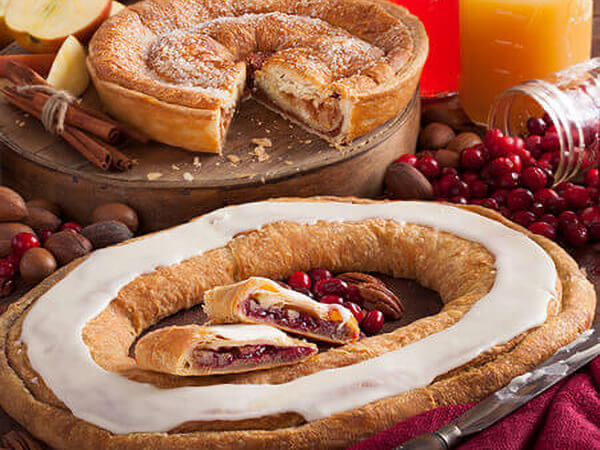This indoor photograph showcases a rustic, cozy table setting against a deep red wall. The wooden table, accented with a red napkin, features a nut and berry mix—predominantly hazelnuts and vibrant red cranberries—spread across the left side. Central to the image is a round pastry, possibly a tart, adorned with white icing. This pastry appears to consist of puff pastry and is filled with cranberries and nuts, likely a mix of pecans and walnuts. In the middle of this pastry ring are fresh cranberries and whole pecans or walnuts.

Behind the pastry, a wooden platter displays a pie, potentially an apple pie, with a visible top and bottom crust and a triangular slice cut out. Accompanying the scene is a jar in the top right corner filled with orange juice, and next to it, another jar tipped over with cranberries spilling out, adding a touch of rustic charm to the overall setting. A knife lies beside the central pastry, ready for serving.